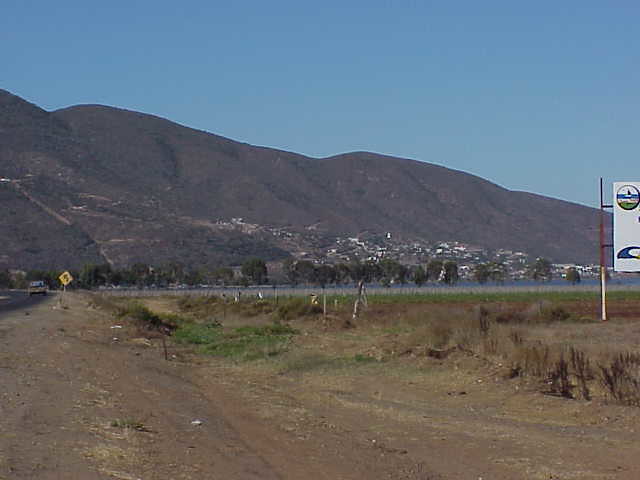The image captures an outdoor setting during midday near a mountain town. The foreground features a muddy and patchy dirt surface, interspersed with patches of grass, weeds, and dead brush. Off to the left side of the image, there is a roadway with a couple of street signs, one being a yellow rectangle with a black arrow pointing left. A light-colored pickup truck can be seen partially behind one of these signs. On the right side, there's a white sign with blue lettering, though the text is too small to read. The midground contains a sizable field predominantly brown with sparse green patches. Distant buildings sit at the foot of a mountain range. The background showcases a mountain, brown and covered with scrub brush, and above it lies a clear blue sky with no clouds. The scene is visually composed of multiple colors including blue, brown, black, yellow, green, and white, reflecting both natural and man-made elements in this serene midday mountain town setting.